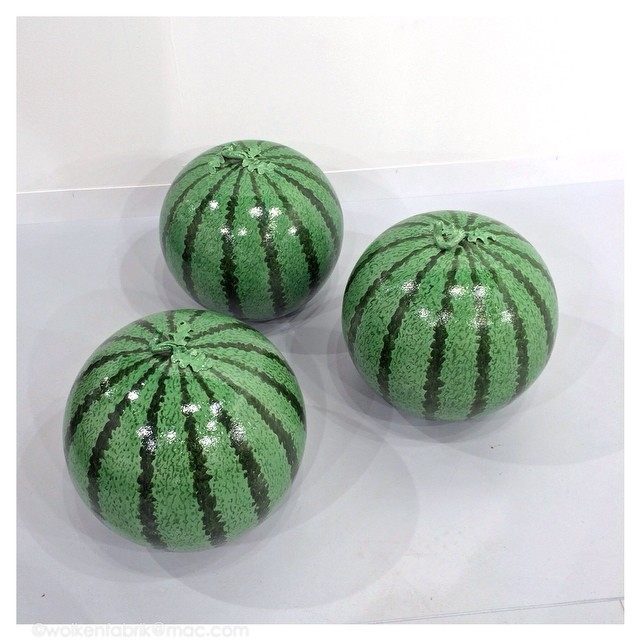This image captures a square-format, color photograph featuring three impeccably round, ceramic watermelons arranged in a triangular pattern on a pristine white surface, against a white background with visible caulking between the surfaces. Each watermelon exhibits a light green skin with darker greenish-black stripes that span from the top, adorned with a ceramic leaf and stem, to the base. The fruit sculptures are notably shiny, reflecting multiple light sources, possibly including a camera flash, and create distinct shadows on the surface below them. These watermelons are exceptionally polished, suggesting they may be display items or have been treated with a reflective finish to enhance their glossy appearance. Their almost lacquered surface contributes to their striking, show-quality perfection.